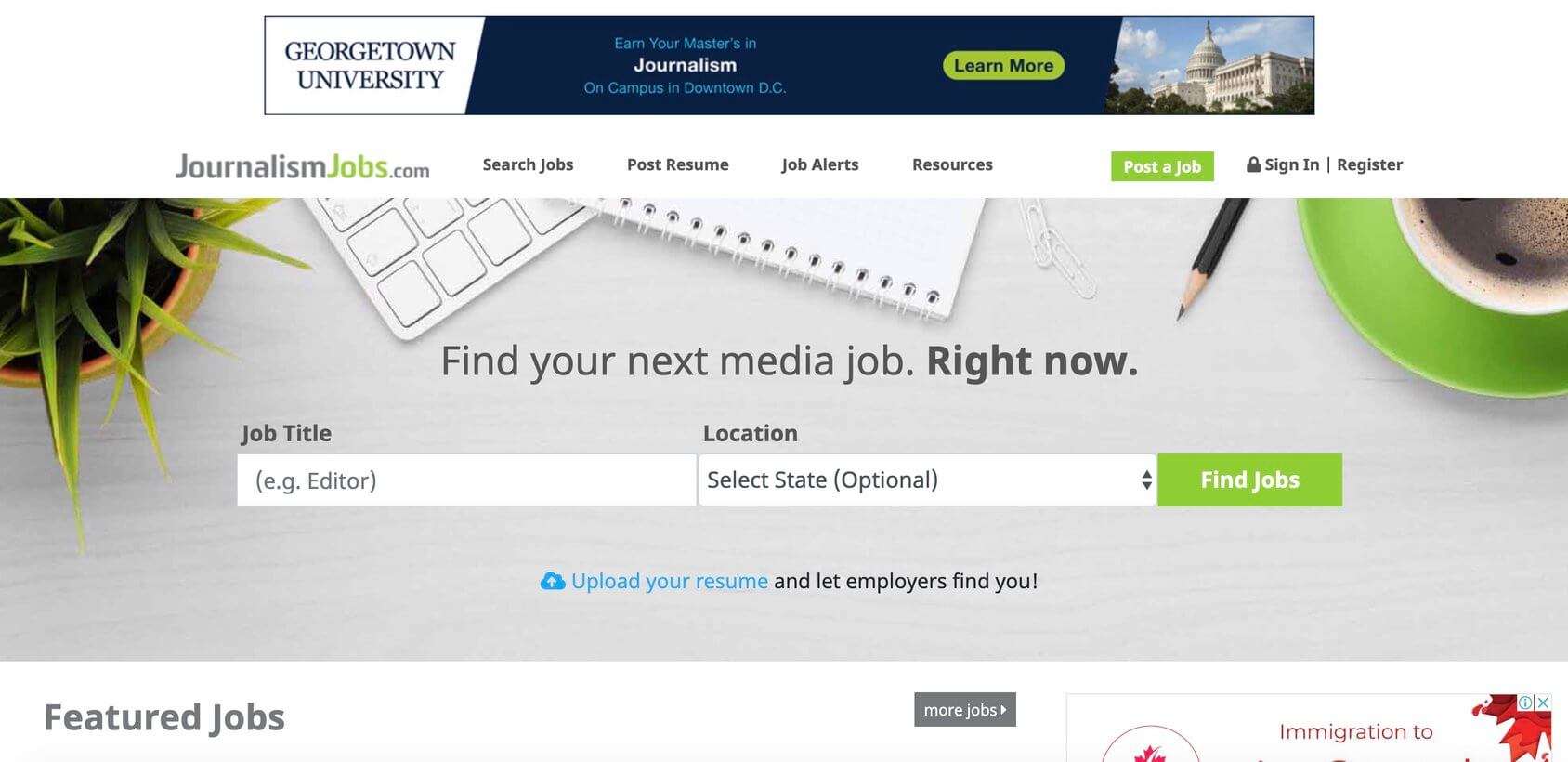Screenshot of the JournalismJobs.com homepage. The horizontal screenshot captures the top navigation menu featuring options such as "Search Jobs," "Post Resume," "Job Alerts," and "Resources." On the right, there are buttons for "Post a Job" and "Sign In/Register." 

Beneath the menu is a large stock photo depicting a neatly arranged desk with a plant, keyboard, notebook, pencil, safety pins, and a cup of coffee. Overlaid on the photo is the text, "Find your next media job right now." 

Below the image, there is a dedicated search function where users can input job titles and locations, with a dropdown to select the state, and a green button labeled "Find Jobs" to initiate the search. To the right of the search function is a section with a cloud icon and the text, "Upload your resume and let employers find you."

Further down, the section titled "Featured Jobs" is visible, but the job listings are cut off. There is also a "More Jobs" button beneath this. To the side, a partially visible Google ad featuring a Canadian maple leaf symbol with the text "Immigration" is also cut off.

At the top of the page, a prominent banner ad for Georgetown University invites users to "Earn your master's in journalism on campus in downtown D.C." The ad includes an image of the Washington D.C. Capitol building and a "Learn More" button.

The overall background of the website is white, giving it a clean and professional look.